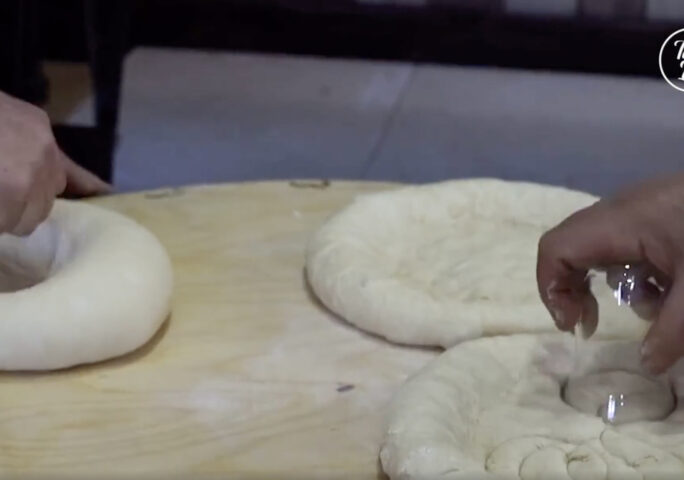The image captures a close-up view of people engaged in bread-making on a wooden table with a brownish-golden hue. On the left side of the table, one person's hand is forming a large ring of dough with a hole in the middle, reminiscent of a bagel or a large doughnut. On the right side, another person's hand is working with a round, thick crust of dough, somewhat resembling a pizza base but too thick to be truly flatbread. This person is using an upside-down glass to cut small, round pieces from the dough. Flour is scattered across the table, indicating active preparation. In the background, there appears to be a gray object, likely a chair, and in the upper right corner, there's a circular design with intricate patterns.